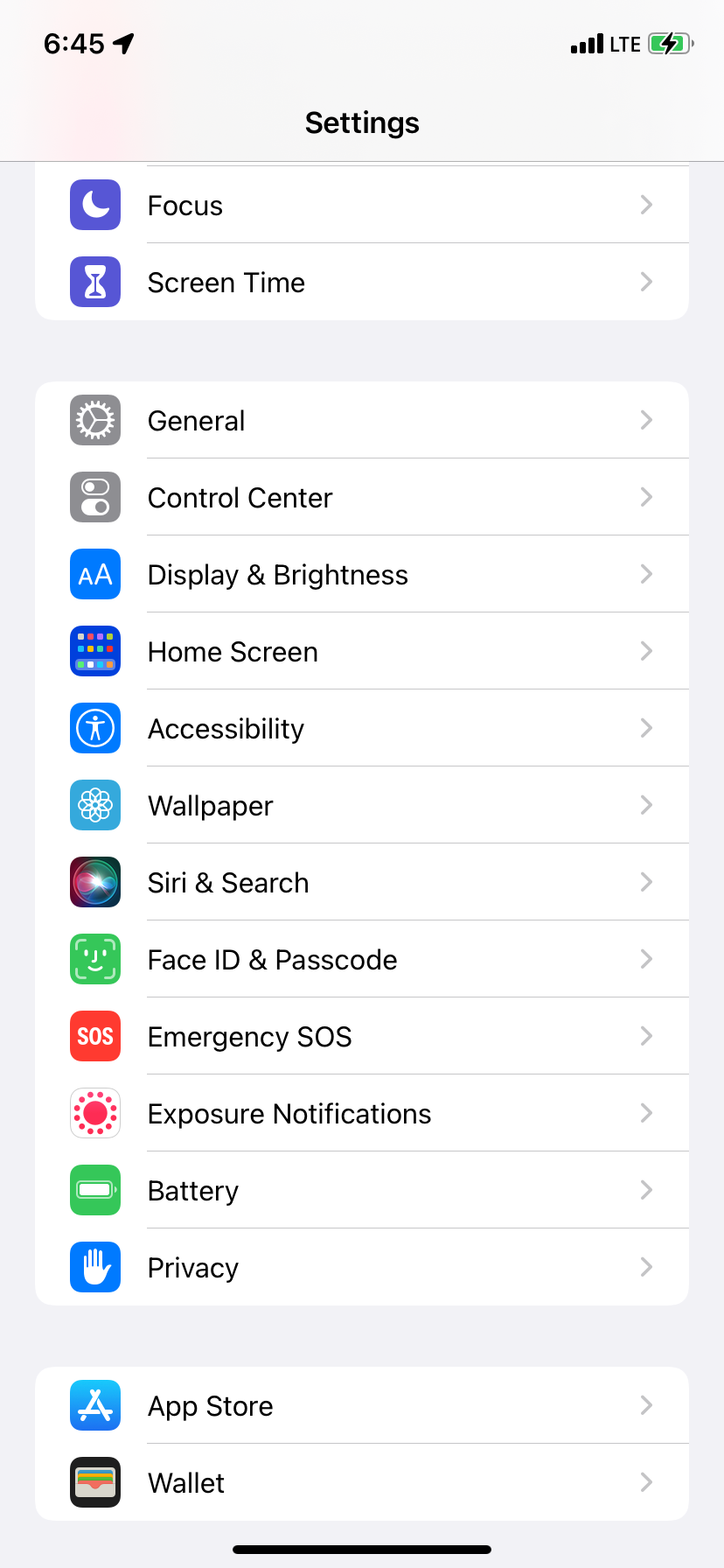This is a detailed screenshot of a phone's settings menu, featuring a clean, white background. At the top-left corner, the time is displayed as 6:45. The top-right corner shows a battery icon nearly full, indicating a 95% charge. 

In the center of the screen is the title "Settings." Below it, the list begins with "Focus Group" and "Screen Time." A light gray divider separates these options from the next section, which includes a comprehensive list of settings categories: 

- General
- Control Center
- Display & Brightness
- Home Screen
- Accessibility
- Wallpaper
- Siri & Search
- Face ID & Passcode
- Emergency SOS
- Exposure Notifications
- Battery
- Privacy

Another light gray divider follows these options, leading to two more selections at the bottom: "App Store" and "Wallet." Each menu option is accompanied by a small arrow pointing to the right, suggesting additional submenus. The very bottom of the screen features a thin black line.